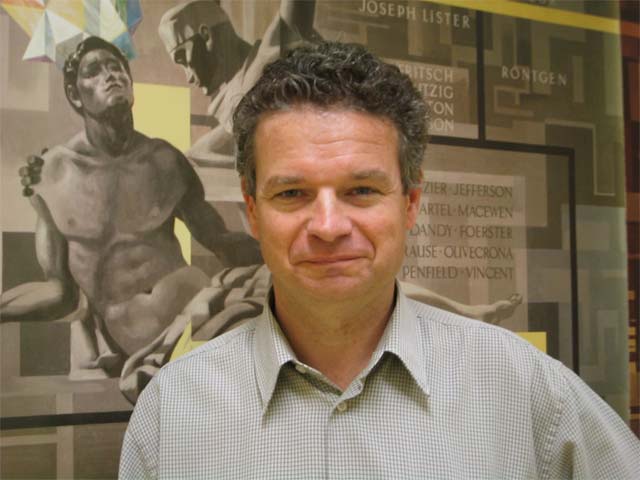The photograph captures a middle-aged white man who is clean-shaven and smiling directly at the camera. He is dressed in a gray shirt adorned with a subtle pattern of small white squares on dark lines, giving it a high-resolution appearance. The focus is on his face and upper body. Behind him, the background features a wall adorned with a large, grayish-black poster filled with names such as Joseph Lister, Ron Egan, Jefferson, MacLean, Forrester, Olive Crona, Winsett, Penfield, Rottgen, McEwen, and Dandy. The poster displays intricate patterns and images that resemble ancient Greek or Roman statues, possibly indicating the setting is a museum. On the left side of the image, more statues, potentially depicting Greek gods, add to the historical ambiance of the scene.